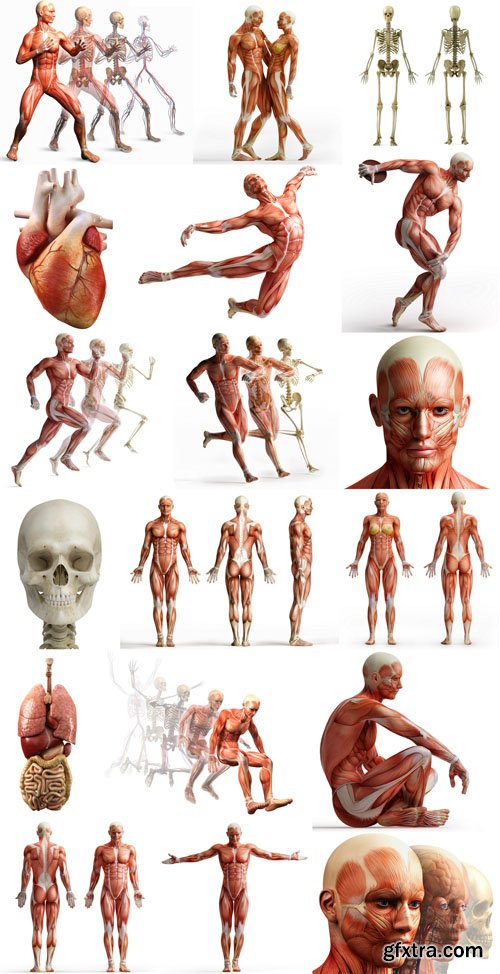This detailed poster, reminiscent of those commonly found in a doctor's office, depicts various anatomical representations of the human body across a six-row by three-column grid. Each of the eighteen sections illustrates either skeletal or muscular anatomy, devoid of natural skin. The depictions range from full human forms in different positions—standing, running, and facing in various directions—to close-ups of specific body parts like the head and the heart. In the top left corner, four skeletal figures are displayed in a row. Another section shows a skeletal figure next to a person who appears to be prancing like a ballerina. Various skeletal and muscular forms are shown, including a figure that looks like it is in a bowling position. The third row includes skeletal muscle figures in a running position and a head with white hair and intense eyes. The next row showcases anatomical details of the heart, lungs, and intestines, along with a series of images that mimic the motion of flipping through a book, showing various movements. Additional sections feature seated figures and those standing with arms outstretched. In the bottom row, forward and backward perspectives are illustrated, including three muscular figures and one skeleton head. The poster includes the letters "GFX Tr a.com".